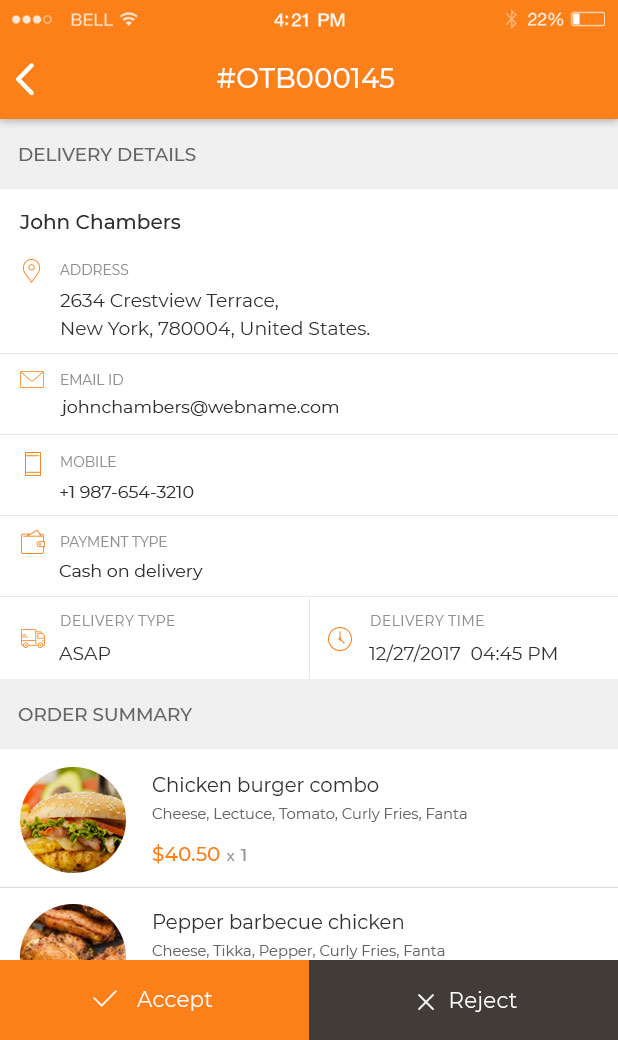The image depicts a screenshot from a food delivery app on a mobile device. 

At the top of the screen, there is an orange banner. On the left side of the banner, there is an icon comprising four small dots, with the dot on the far right being unfilled. Adjacent to this is the text "Bell", followed by the cellular signal strength indicator. Centrally positioned at the top, the time is displayed as 4:21 p.m. On the right side, there are icons for Bluetooth and the battery life indicator, showing 22% remaining battery.

Below this, a navigation banner includes a back arrow, with the text "Order Number OTB000145" centered within it. 

The main content area of the screenshot contains detailed delivery information as follows:
- "Delivery details"
- "John Chambers"
- "2634 Crestview Terrace, New York, 78004, United States"
- "Email ID: johnchambers@webname.com"
- "Mobile: 1-987-654-3210"
- "Payment type: Cash on Delivery"
- "Delivery type: ASAP"
- "Delivery time: 12-27-2017, 4:45 p.m."

An "Order Summary" section lists the ordered items and their prices:
- "Chicken Burger Combo" includes cheese, lettuce, tomato, curly fries, and Fanta, priced at $40.50 (quantity: 1)
- "Pepper Barbecue Chicken" includes chicken tikka, pepper, curly fries, and Fanta, but the remainder of this item’s details are cut off.

At the bottom of the screen, there are two buttons: an orange "Accept" button with a check mark on the left, and a black "Reject" button with an 'X' mark on the right.